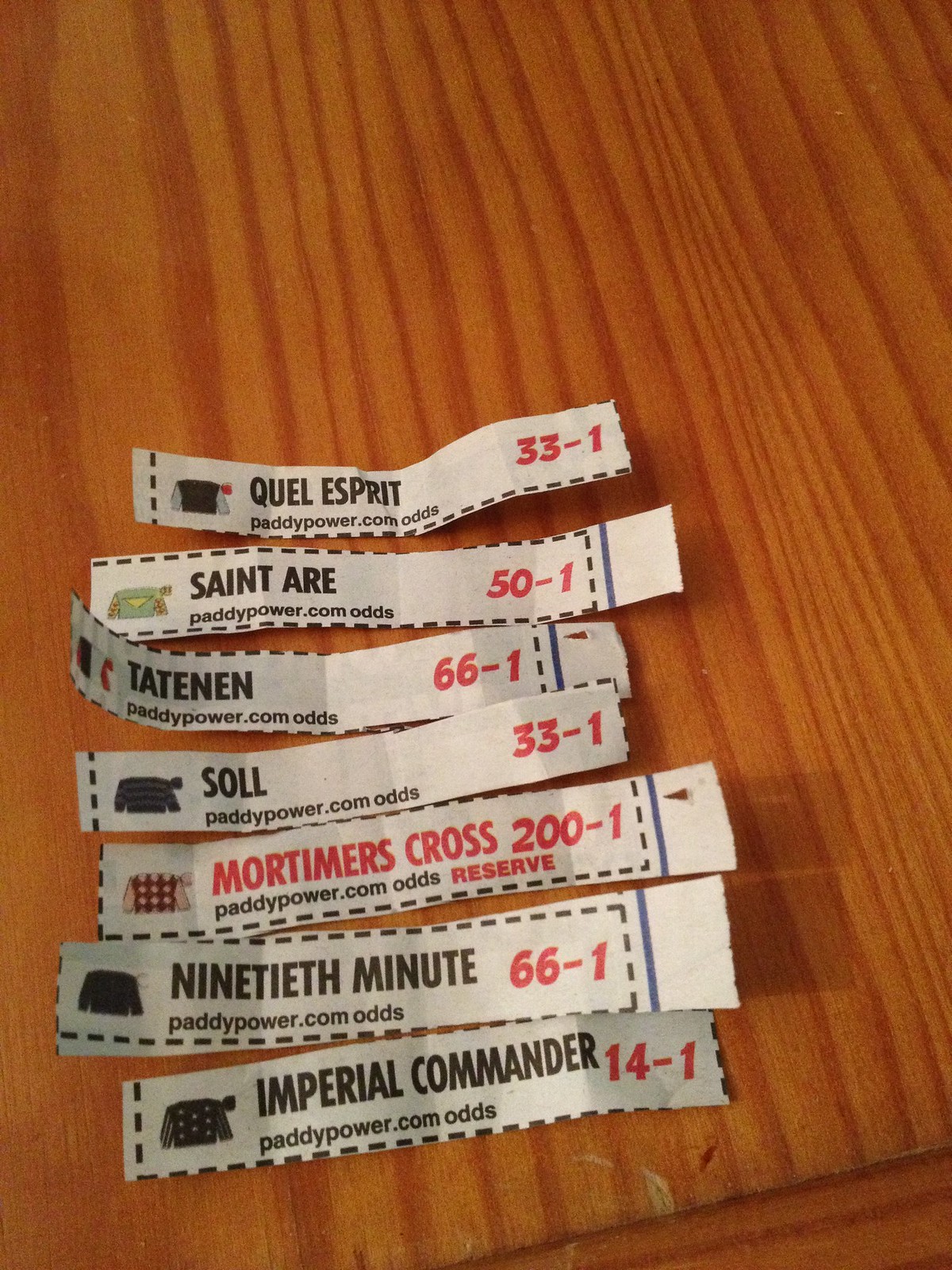This image features a wooden tabletop with a yellowish golden hue and distinct brown wood grain. Seven small slips of paper, seemingly cut out from a newspaper, are spread out on the table. These slips likely represent betting tickets from a horse race, given their format and content. Each slip includes a jockey's illustrated kit on the left, a horse's name in capital letters in the center, and the betting odds in red on the right. The information on the slips reads as follows: 

1. "Quill Coel Esprit" with odds of 33-1.
2. "St. Air" with odds of 50-1.
3. "Taitnen" (with a possible spelling variation "Tatemenen") with odds of 66-1.
4. "Sol" with odds of 33-1.
5. "Mortimer Cross" with odds of 200-1.
6. "90th Minute" with odds of 66-1.
7. "Imperial Commander" with odds of 14-1.

All slips also feature the text "PaddyPower.com Odds" in black beneath the horse’s name, indicating the source of the bets.